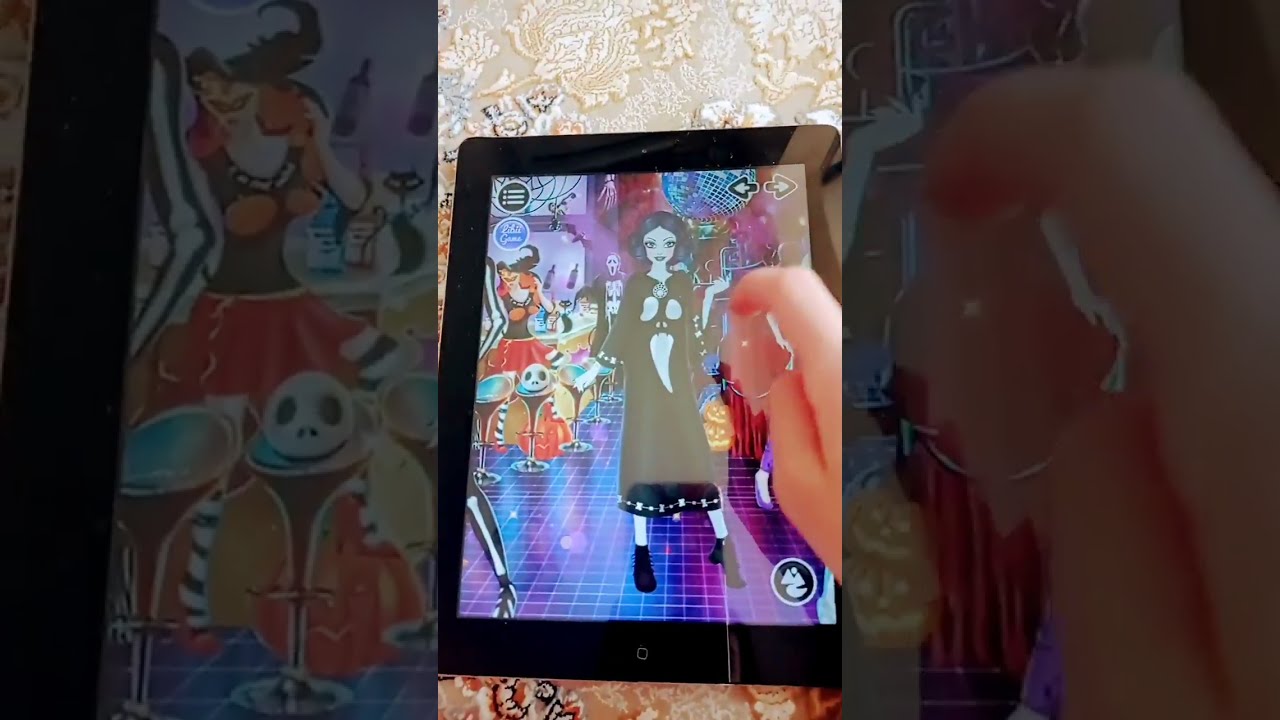In the center of this wide rectangular image, a photograph of an iPad is displayed in portrait orientation on a tan and gold embroidered floral-patterned surface. The iPad, with its thick black frame and prominent square button at the bottom, appears to be of an older model. The screen of the iPad shows a game featuring a gothic-themed character—a tall woman with pale skin, short black hair framing her face, and a long black dress ending at her shins, paired with black boots. She stands on a shiny blue and purple checkered floor, dotted with small square tiles. A disco ball hangs above her, adding to the scene's motif. Off to the side, there is another character wearing a red dress, a witch hat, and a bra made of pumpkin shapes, reinforcing the Halloween theme. A human hand is visible on the right side of the image, seemingly swiping across the screen.